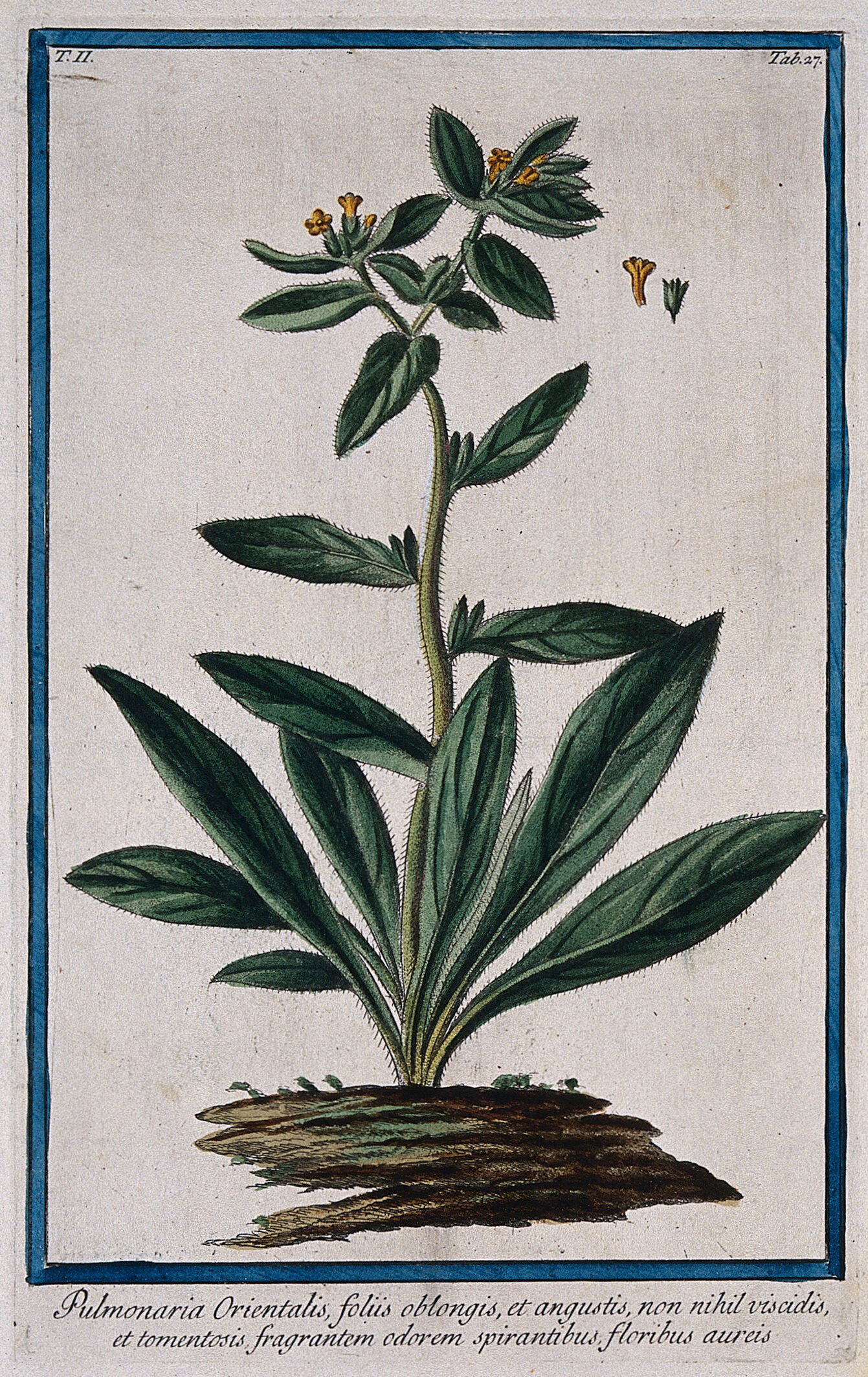This detailed botanical illustration features a hand-drawn plant, painted on a canvas with a cream-colored background. The artwork is bordered by a thin, turquoise frame, set within a wider blue border that leaves some space between the edge and the artwork itself. In the upper left-hand corner, a watermark reading "T. II." is visible, while the upper right-hand corner is marked with "tab 27."

The main subject of the painting is a dark green plant with a thick, fuzzy stem and wide, basil-like leaves. The plant grows from a small patch of dirt depicted at the bottom of the image, which only occupies about a third of the canvas base. The leaves cluster more densely at the base and become smaller as they ascend along the stalk. At the very top, the plant bears yellowy-orange and blue flowers, their stamen and pistil distinctly visible.

Near the bottom of the painting, there is a cursive inscription in what appears to be Latin, reading: "Pulmonaria orientalis folius oblongus et angustus non neal vicidius." This detailed and meticulously rendered image conveys not only the botanical complexity of the plant but also an artistic beauty, combining scientific observation with the aesthetic qualities of fine art.